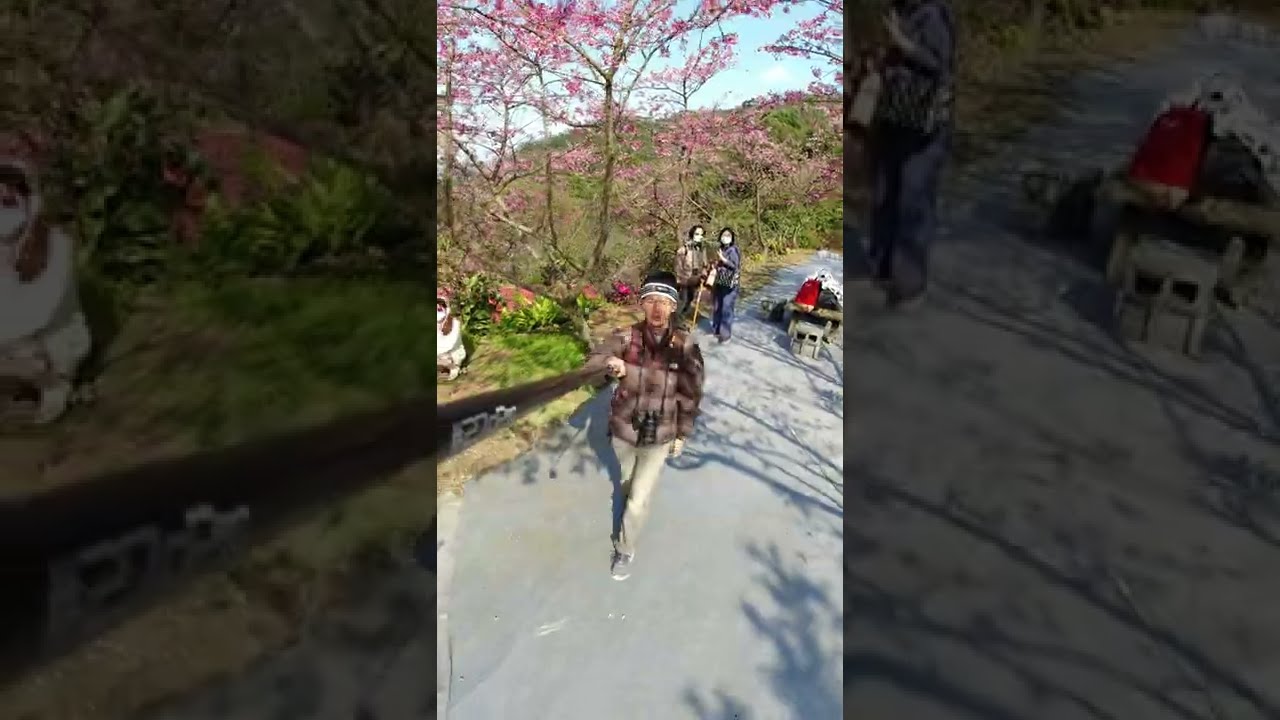The image consists of three panels, with the main picture centered and flanked by darkened versions of the left and right sections of the main image. It depicts a walking trail in a park, adorned with trees bearing purple and pink leaves, suggesting a spring setting. A man is walking directly toward the camera, dressed in tan slacks, a brown checkered jacket, and a blue and white cap. His right arm is raised as if checking his watch, and he is wearing gray shoes. A camera dangles from his neck, and he appears to be taking a selfie with a photostick. Behind him are two women in jackets wearing COVID masks. To the right side of the trail, there's an ambiguous object that might be a red-topped table or bench. A hill with more trees is visible in the background. The primary colors in the image are pink, green, white, and blue, contributing to a vibrant spring atmosphere.